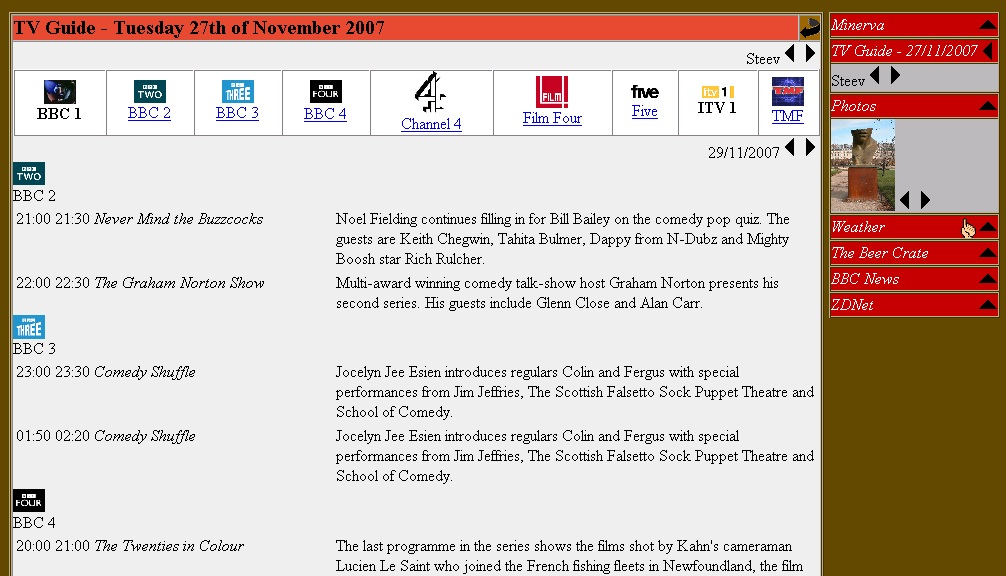This is a detailed caption for the screenshot you described:

---

This screenshot captures a detailed view of a TV guide from Tuesday, November 27th, 2007. At the top, a prominent red menu bar displays the date and the title "TV Guide." Below the bar, there is a comprehensive list of channels, each represented with its respective logo: BBC 1, BBC 2, BBC 3, BBC 4, Channel 4, Film 4, 5, ITV 1, and TMF. Notably, most of these channel listings feature clickable links, though BBC 1 and ITV 1 are exceptions without links.

Directly beneath this list, the guide reiterates the date, "29-11-2007," accompanied by navigational arrows suggesting the ability to browse different dates. The main content below showcases the schedule of television programs, starting with BBC 2, which lists shows such as "Never Mind the Bullocks" and "The Graham Norton Show," including detailed descriptions and guest information for each show.

Following BBC 2, the guide lists BBC 3's schedule, featuring two episodes of "Comedy Shuffle." The entries appear peculiar as they list identical guests at different times. BBC 4 is also featured, with an entry for a program titled "The 20s in Color."

Occupying approximately 20% of the right-hand side of the page, there's a dropdown menu for selecting the TV guide date. Below this, the name "Steve," spelled "S-T-E-V," is visible, possibly indicating user-specific preferences or customizable guides. The page also includes sections for photos, weather updates, "The Beer Crate," BBC News, and ZDNet, which may represent favorited content or additional features of the TV guide.

---

This detailed caption provides a thorough description of the screenshot, capturing all the key elements and potential functionalities as described.